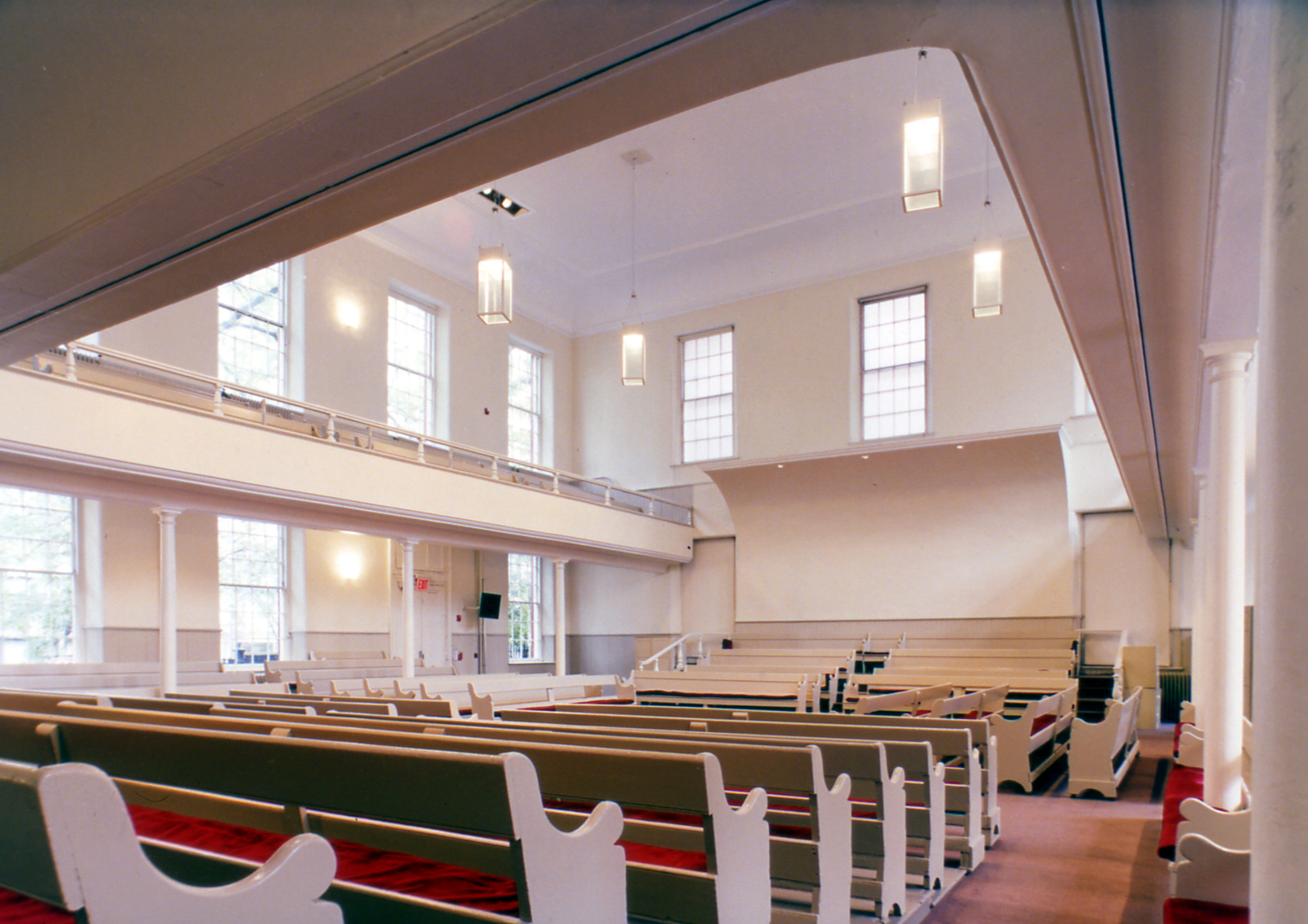This photograph captures the interior of a modern-style church characterized by its high, flat white ceilings adorned with multiple rectangular white lights. The space is lit by both natural light streaming through large windows situated both at the top and bottom levels and artificial lighting. The church features a second-floor balcony area to the left, enclosed by white fencing, which houses wooden bleachers and is supported by white columns.

On the ground floor, there are approximately eight rows of light brown benches, each equipped with red-cushioned kneelers at the front. The arrangement of the seating is such that all benches face towards the center of the room, giving it an intimate and inclusive atmosphere. The décor is minimalist, with an emphasis on white surfaces and a few small, modernist touches, including a subtle cross in the background. The overall aesthetic is clean and contemporary, with no visible text or people present in the image, allowing for a serene and contemplative environment.